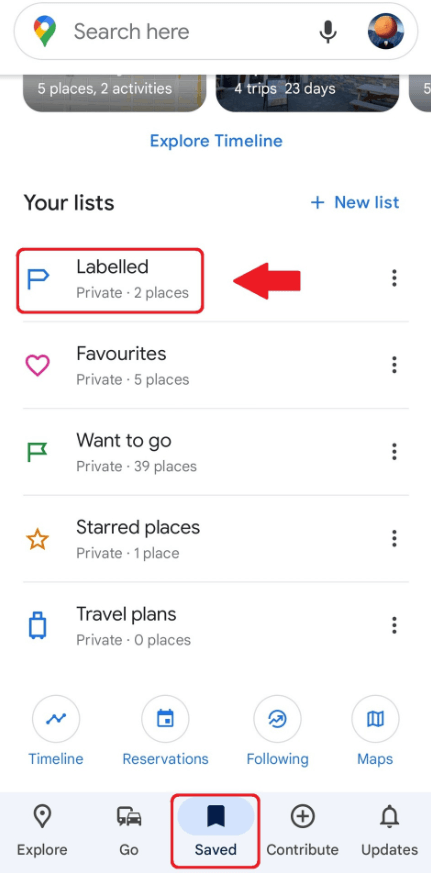This is a detailed screenshot of the Google search app interface. At the top of the screen, a Google logo in the shape of a pin drop is prominently displayed. To its right, the phrase "Search here" is written in light gray letters within a search bar. On the far right of the search bar, there is a microphone icon and a circular profile picture. Below the search bar, the page scrolls down to display partial bottoms of three thumbnails. The first thumbnail's text reads "Five places, Two activities" in white font. The second thumbnail says "Four trips, 23 days." The third thumbnail shows only the number "5" in the far right corner of the screen. Beneath this section, the phrase "Explore Timeline" appears centered at the top of the next segment of the page in blue font. To the left, in bold black letters, it says "Your Lists," under which a section labeled "Labeled" is highlighted with a red box and pointed to by a red arrow. At the very bottom of the screenshot, the word "Saved" is encapsulated in another red box.